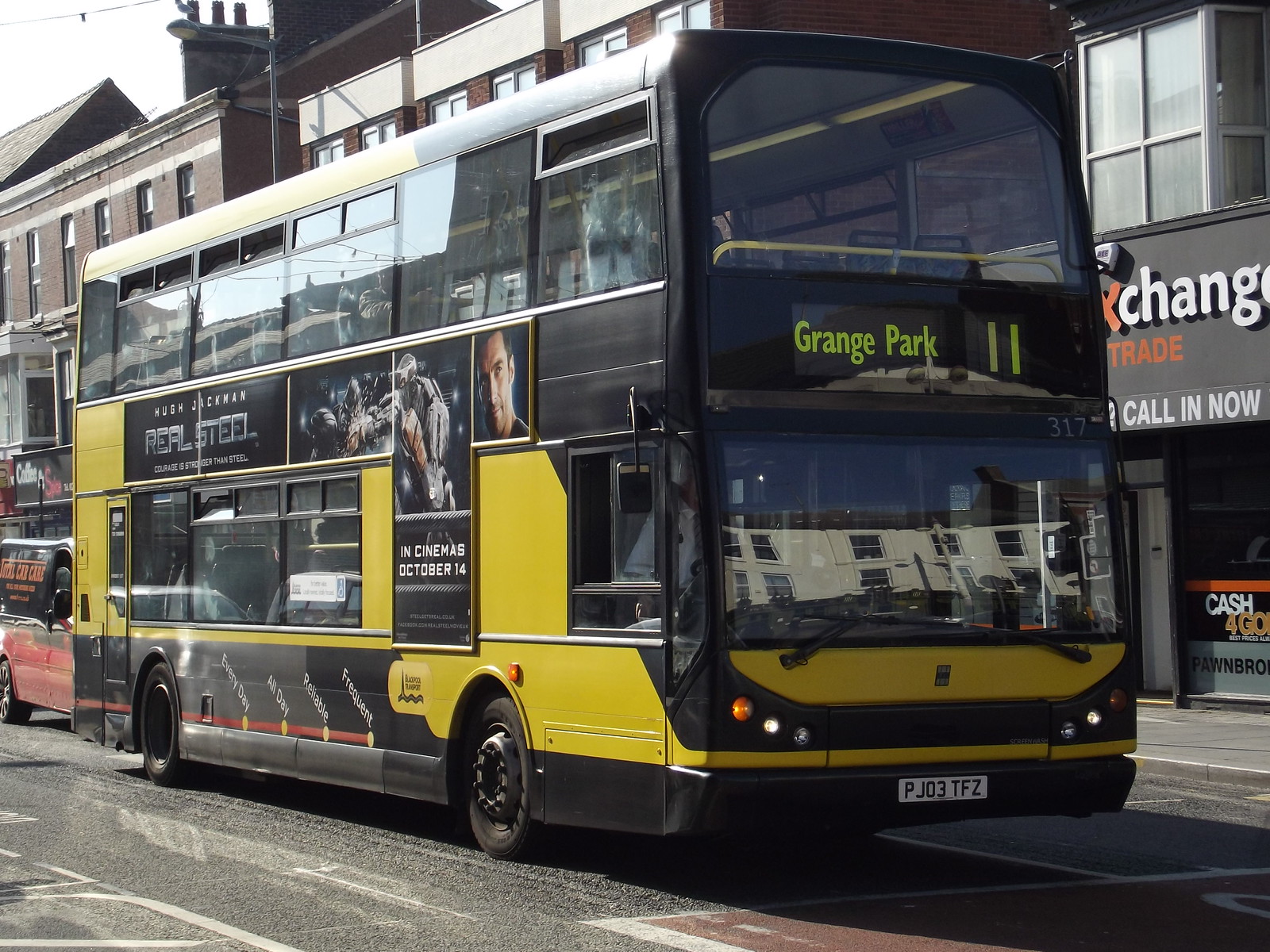This image captures a bustling street scene in a town with a vibrant double-decker public bus as the focal point. The bus, predominantly black with striking yellow designs and patterns, features several colorful posters. Its glass windows reflect the surroundings, adding depth to the image. The vehicle's registration number, PJO3 TFZ, is visible on the bumper, above which are the headlights and dipper lights on either side.

The main windshield showcases a reflection of the building opposite, accentuated by the large wipers. A digital display between the upper and lower decks reads "Grange Park 11," indicating its route. The lower portion houses the driver's section, and on the top right corner of the bus, the number 317 is prominently displayed.

A vivid movie poster of "Real Steel" adorns the side of the bus, featuring the title and tagline: "Real Steel, Hugh Jackman, Courage is Stronger than Steel, in cinemas October 14." Below the passenger windows, another poster reads: "Frequent, Reliable, All Day, Every Day," nestled between the two tires.

Behind the bus, a small truck is partially visible, adding to the dynamic urban scene. The background reveals a series of buildings with shopfronts, one of which has signage that reads: "Exchange, Trade, Call-In Now," along with another shop bearing the words "Cash, 4, Go, Pawn Bro." The road beneath the bus is clearly visible, grounding the scene in a typical town setting.